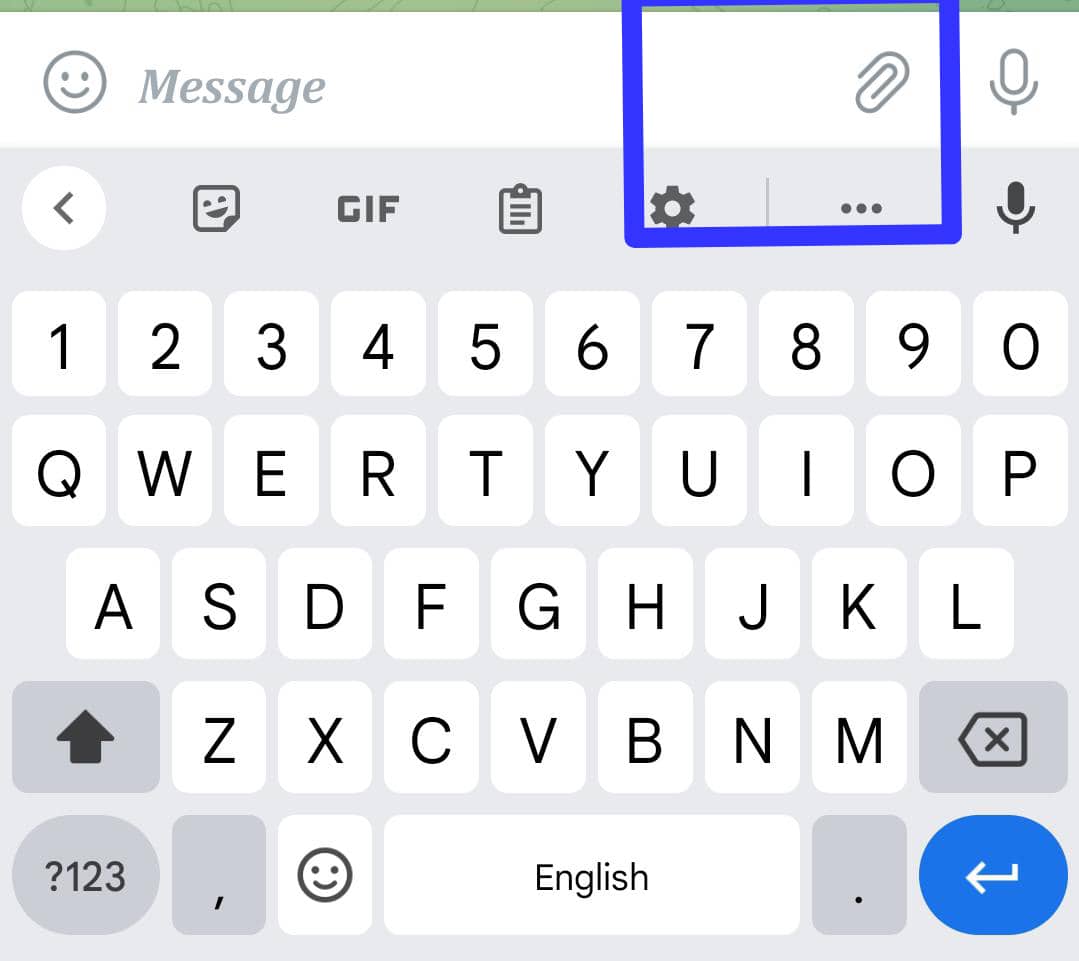This is a detailed screenshot of an enlarged smartphone screen interface, specifically showcasing the mobile on-screen keyboard. At the top of the screen, there is a smiley face icon, followed by a message bubble, both presented clearly. Below this, the interface features a blue action bar containing several utility icons including a settings wheel, three vertical dots, and a paperclip icon. Adjacent to this bar, on the right, are two microphone icons; one directly to the right of the blue bar and another positioned below it.

Moving leftward from the bottom microphone icon, the toolbar displays additional icons: a document icon, a GIF icon, a sticker icon, and a left-facing arrow enclosed in a white box. Below this toolbar, the on-screen keyboard is visible with its typical layout and gray function buttons, such as the comma, period, question mark, number switch (123), backspace, and shift. On the extreme right of the keyboard, there is also another left-facing arrow icon within a blue box. This clarifies that the image displays a virtual keyboard projected on the smartphone screen, not a physical keyboard, emphasizing its versatility for on-screen use.